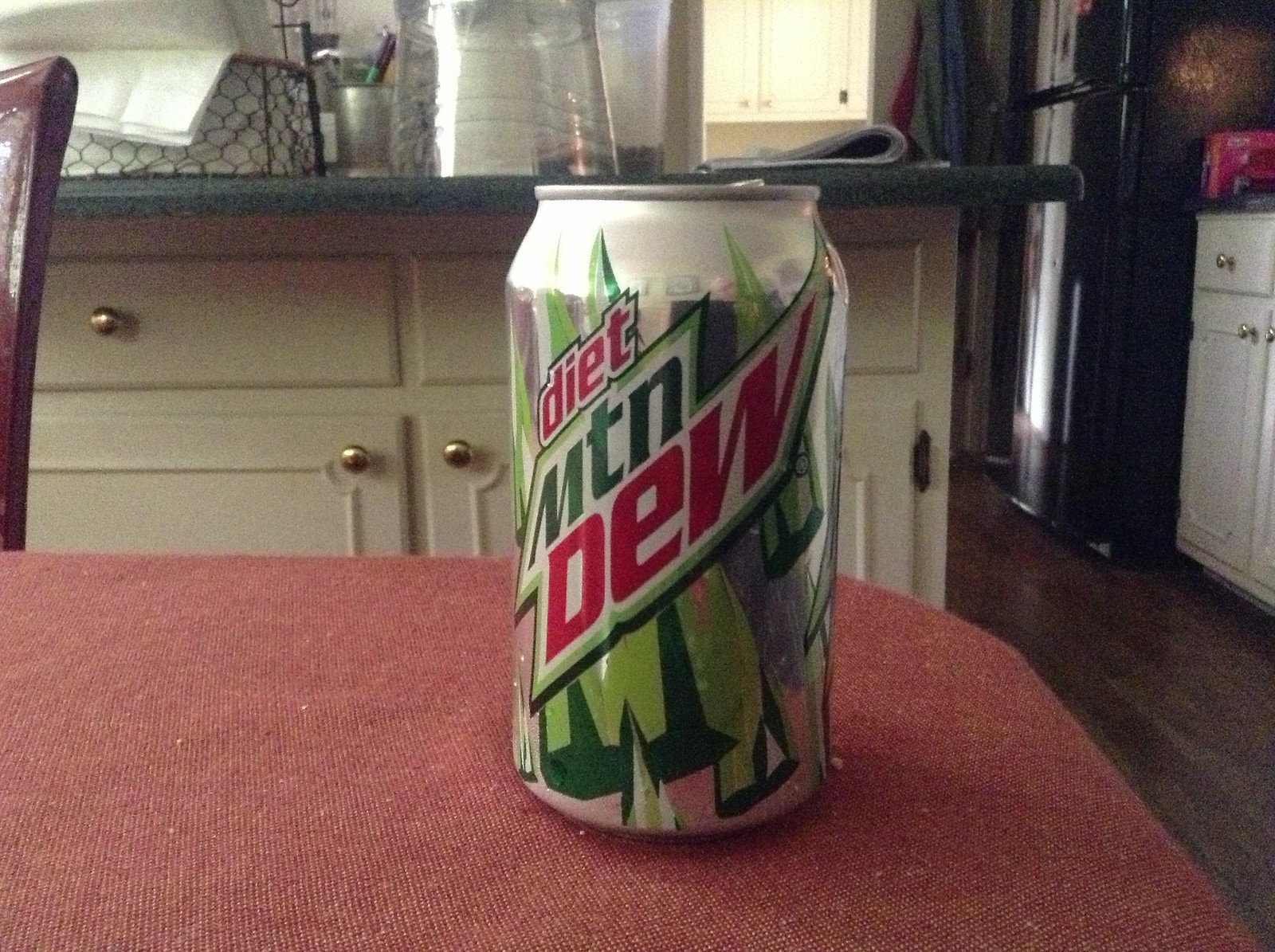This photograph features a Diet Mountain Dew aluminum can prominently placed on the rounded corner of a table adorned with a maroon tablecloth. The can, boasting a silver exterior, displays the Mountain Dew logo in bold red and dark green colors set against a white background, with an array of green, spiky designs embellishing the area around the logo. In the background, white cabinets with stainless steel hardware and a blue countertop are visible. The countertop holds various items: a wire basket, a stainless steel cup containing pens, some inverted glassware, and a rolled-up newspaper. To the right of the image, a dark brown wooden floor is partially seen, along with additional white cabinetry and a dark refrigerator-freezer unit situated in the far background.